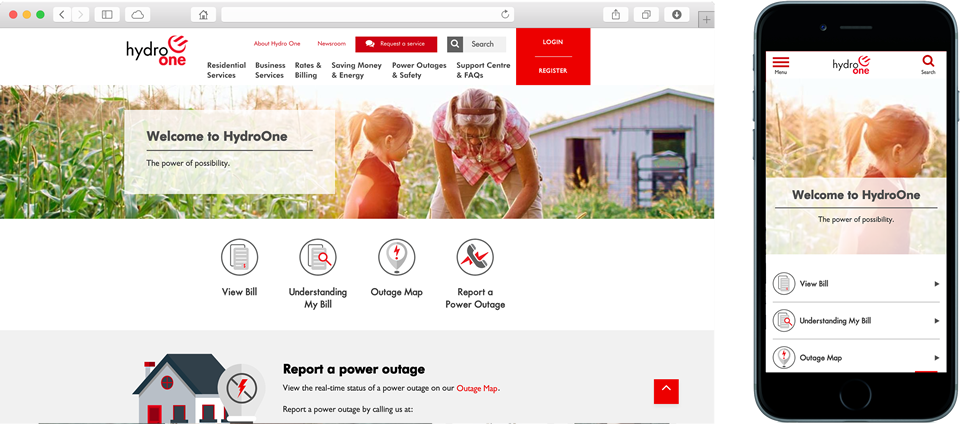The image showcases both the desktop and mobile versions of the Hydro One website, viewed on a MacOS using Safari. The desktop version prominently features a welcoming message: "Welcome to Hydro One, the power of possibility." The background image captures a serene scene of a young girl and her grandmother tending to a lush cornfield, with a rustic shed in the background. Grandma is engaged in some activity while the girl observes. The top navigation includes links to various sections such as Residential Services, Rates and Billing, and Power Outages, indicating that Hydro One provides essential utilities, possibly electricity generated through hydropower. Additional features mentioned include options to report power outages, view real-time outage statuses, and report an outage via a provided phone number. The mobile version on the right mirrors the desktop layout in a compact form, ensuring ease of access across devices. An iPhone mockup is used to display the mobile interface.